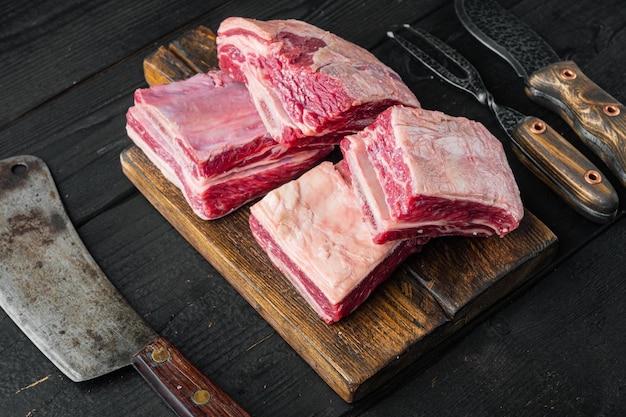On a rough, black wooden surface, likely part of an outdoor setting, rests a rugged, dark brown butcher block-style cutting board. Arranged carefully on the board are four slabs of raw beef, each displaying vivid layers of bright red meat marbled with white fat, hinting at their freshness and direct cut from the animal. To the left of the cutting board, an antique cleaver with a distressed steel blade bearing black and brown marks lies, its handle crafted from wood. On the right side, an old two-prong fork with a medium brown handle and a gunmetal gray blade shares space with a curved knife of similar aged appearance, both tools having pockmarked, blackened metal and wooden handles. The scene evokes a sense of rustic culinary preparation.